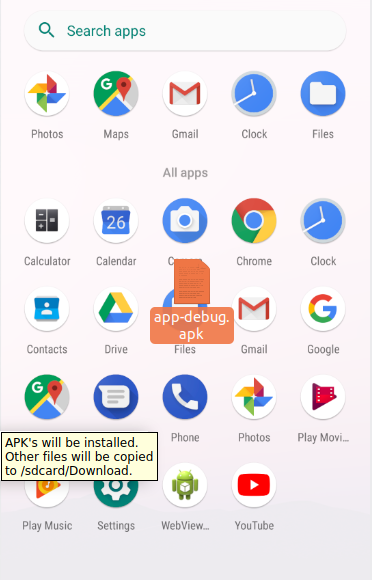In the image, there is a screenshot of a smartphone's home screen showcasing a variety of app icons organized in a grid layout. At the very top, there's a search bar with green text on a white background that reads "Search apps." Directly below, several popular app icons are visible:

- **Top Row (from left to right):** 
  - **Photos:** The first icon, accompanied by text, indicates the Photos app.
  - **Maps:** The second icon represents the Maps app.
  - **Gmail:** Next is the Gmail app icon.
  - **Clock:** Followed by the Clock app icon.
  - **Files:** The last icon in the top row is Files.

Below this top row, there is a section labeled "All apps," followed by another assortment of app icons:

- **Second Row (from left to right):**
  - **Calculator:** The first icon is for the Calculator app.
  - **Calendar:** Next, the Calendar app icon.
  - **Camera:** Then the Camera app icon.
  - **Chrome:** Followed by the Chrome browser icon.
  - **Clock:** Again, the Clock app icon appears.
  - **Contacts:** Then the Contacts app icon.
  - **Drive:** Next to it is the Drive app icon.
  - **Files:** Below this row, there's another Files app icon, but this one has an overlapping open app or widget labeled "app debug APK."

Continuing with the visible apps:
- **Third Row (from left to right):**
  - **Gmail:** Another instance of the Gmail app icon.
  - **Google:** The icon for the main Google app.
  - **Google Maps:** The Google Maps app icon.
  - **Messaging:** Next is the Messaging app icon.
  - **Phone:** The Phone app icon.
  - **Photos:** Followed by another Photos app icon.
  - **Google Play Movies:** The icon for Google Play Movies.
  - **Google Play Music:** The icon for Google Play Music.
  - **Settings:** The Settings app icon.
  - **Web View:** The Web View app icon.
  - **YouTube:** Finally, the YouTube app icon.

Additionally, there is a pop-up box at the bottom which reads: "APKs will be installed. Other files will be copied to SD card/download."

This detailed view highlights the organization and the selection of apps available on the smartphone, featuring both essential and popular utility applications.